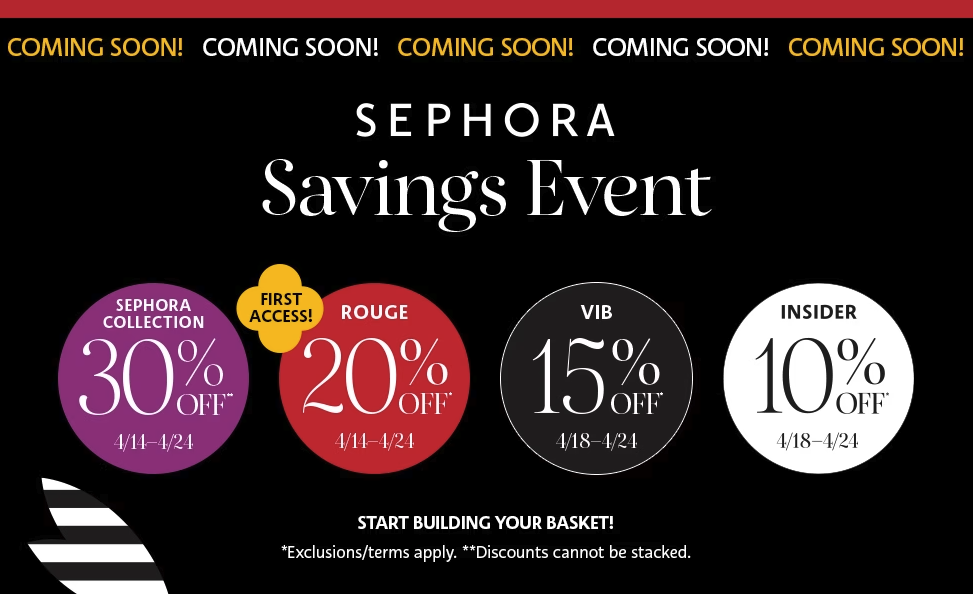The promotional image features a vibrant and dynamic layout, primarily centered around Sephora’s upcoming Savings Event. 

In the top left corner, alternating yellow and white text repeatedly displays the phrase "Come and Soon," creating a sense of urgency and anticipation. Dominating the central portion of the image is large, bold text reading "Sephora Savings Event," ensuring immediate recognition of the brand and the event.

On the left side of the image, a prominent purple circle contains a text that reads "Sephora Collection 30%," along with the dates "4/14 - 4/24." This indicates a special offer on Sephora Collection items during the event period.

To the right of this, a large red circle announces "Rouge 20% Off," also valid from "4/14 - 4/24." Below this, a gray circle indicates "V.I.B. 15% Off," and a white circle reads "Insider 10% Off," all with the same event dates clearly noted.

A yellow, flower-like symbol appears next to the red circle, adding a decorative touch. In the lower part of the image, a message encourages customers to "Start building your basket," but it also notes that "Star exclusions/terms apply" and emphasizes that "Discounts cannot be stopped."

The background is predominantly black, which makes the colorful text and symbols stand out more vividly. The bottom part of the image alternates with white and black spaces, adding to the dynamic and engaging design.

In the top right corner, a bright red bar with multiple exclamation marks ("!!!!") draws additional attention, creating a final touch of excitement about the event.